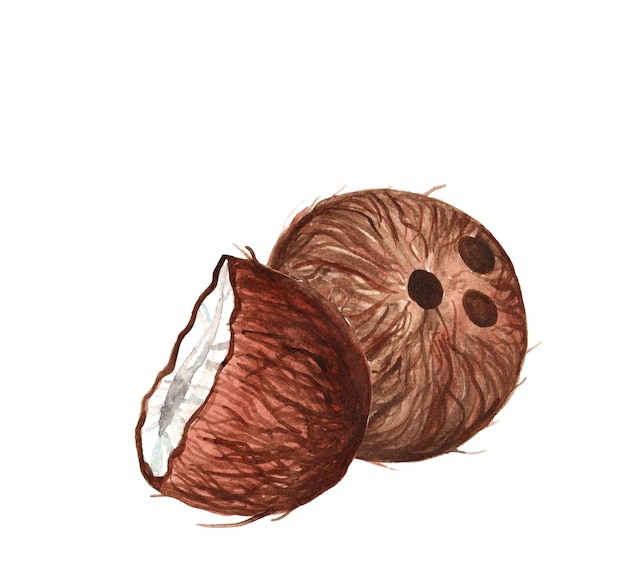This detailed illustration on a solid white background features two coconuts, rendered using either marker or paint. In the foreground is a half coconut with jagged, broken edges, revealing its thick white meat encased in a dark, fibrous, hairy shell. Thin brush strokes are visible throughout, emphasizing the textural disparity between the smooth interior and the rough exterior. The coconut displays a spectrum of browns, from dark to reddish hues. Behind it, a whole coconut stands, exhibiting the characteristic three holes at the top, reminiscent of a bowling ball. This intact coconut also showcases a similar fibrous texture, with thin, stringy brown fibers covering its surface, varying from medium to light brown. The attention to detail in the brushwork highlights the natural textures and colors of the coconuts, creating a striking contrast against the plain backdrop.